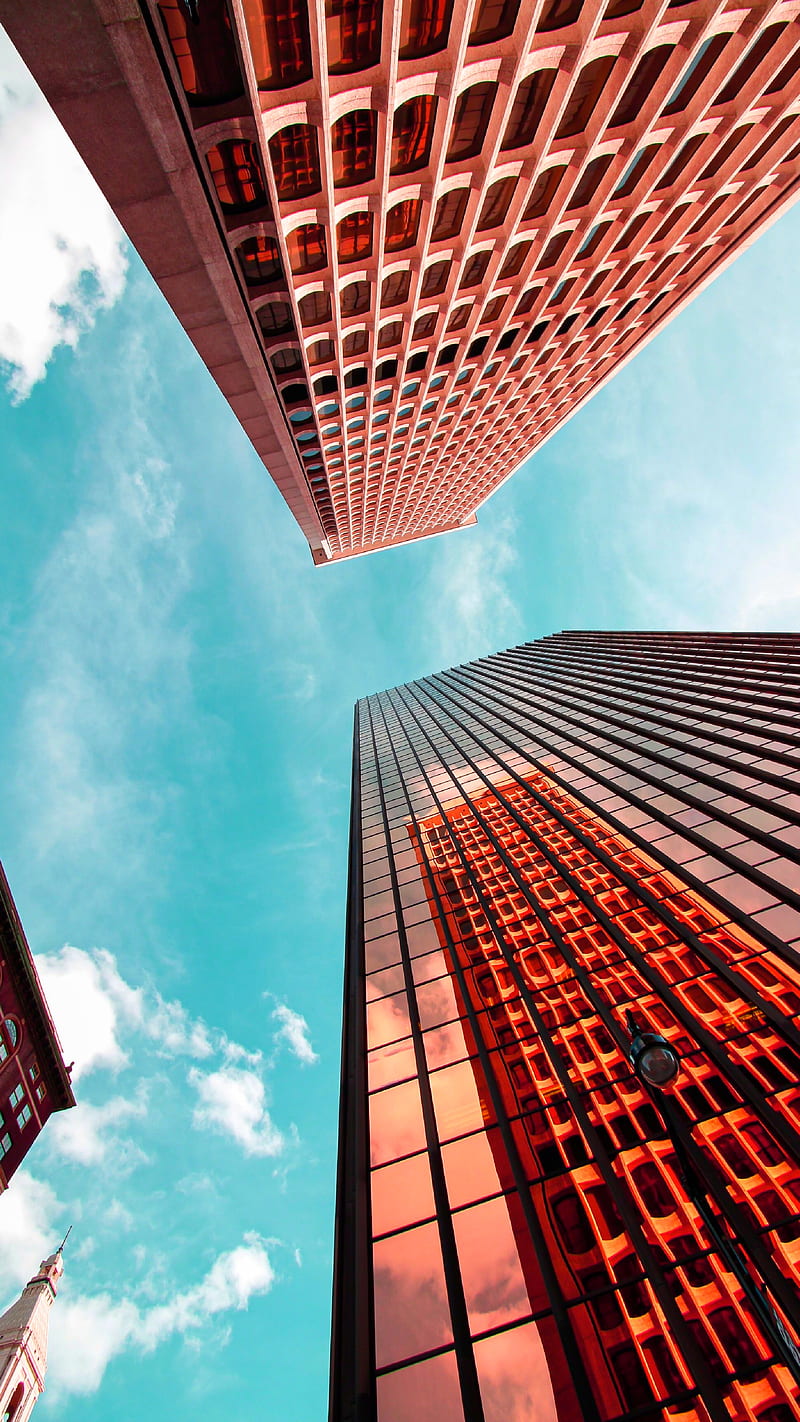The image captures a stunning upward perspective from the street, focusing on two towering skyscrapers that dominate the scene. Both structures exhibit a highly reflective orangey-brown glass facade, mirroring the surrounding elements and sky. The sky itself is a brilliant light blue, almost turquoise, dotted with passing white clouds, indicating a bright, clear day. The skyscraper on the lower right-hand side is nearly enveloped in glass, showcasing reflections of orangey clouds and nearby structures, including a streetlamp. Meanwhile, the skyscraper descending from the upper part of the image reveals numerous window openings. Poking out from the left side of the frame are glimpses of another building and a distinctive white steeple, reminiscent of a clock tower or church spire. Together, these elements create a rich, dynamic composition that conveys the height and architectural grandeur of an urban skyline.